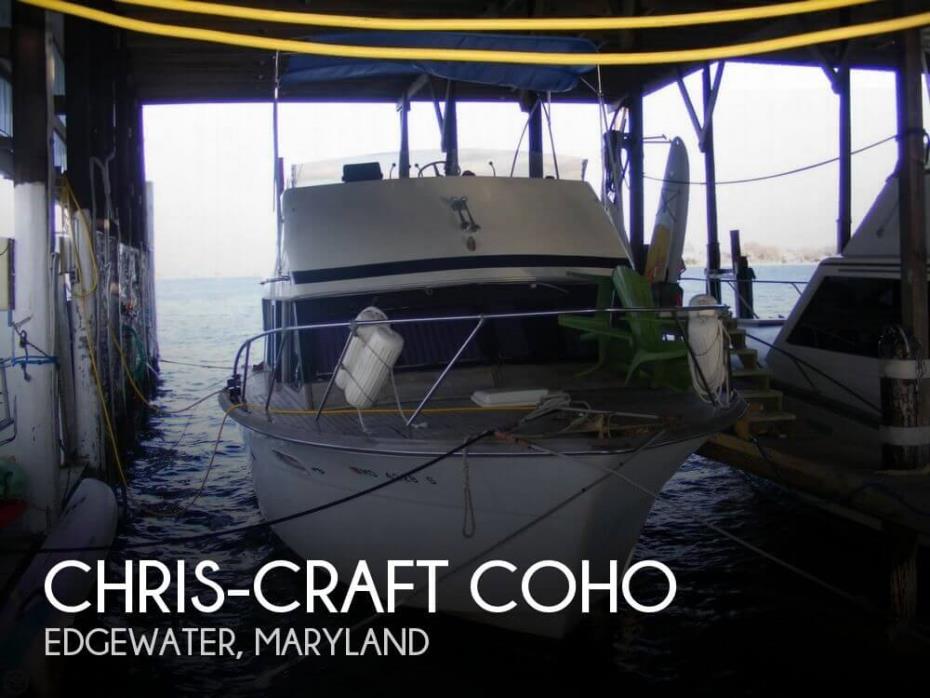The image features a small motorboat from the brand Chris Craft, specifically the "Chris Craft Coho," docked in an outdoor dockyard. The boat is primarily white with fiberglass construction and a silver metal railing around the front. It has a prominent window on the top front, and above that, an open-air deck with a blue awning. The boat is situated in an open shed-like structure that resembles a ship garage, with tall metal poles and walls painted white halfway up, transitioning to a dark brown color. 

The boat is tied to the dock with several yellow and black ropes. At the boat’s bow, there's a stack of green lawn chairs. On the right side, partly visible, there seems to be another white boat. The upper left-hand corner of the image displays the text "Chris Craft Coho, Edgewater, Maryland" in large white letters. Additional objects like a surfboard and two roundish lifeboats can be seen on the boat. The scene has water visible both directly beneath and behind the boat, with a hint of landscape in the distance. The overall atmosphere is somewhat dim, suggesting the structure provides partial shade.